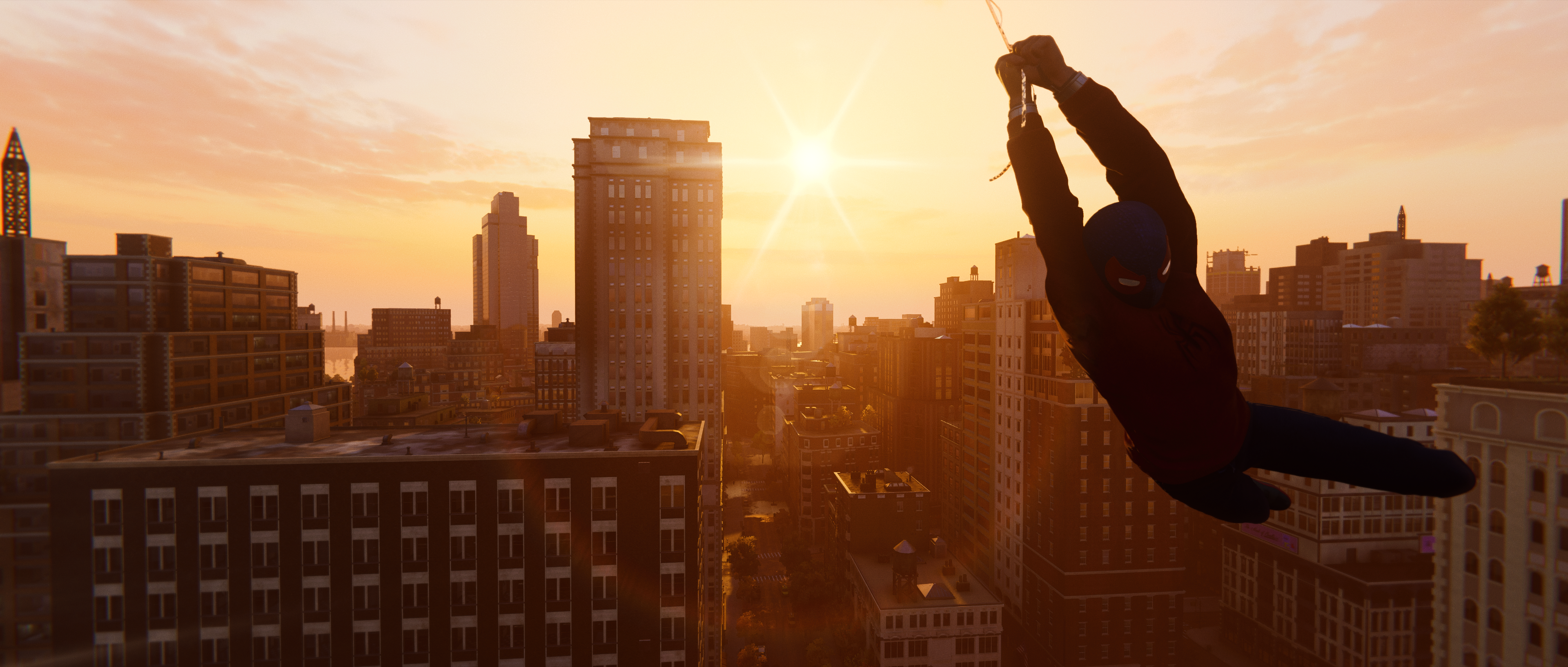In this animated scene, likely from a video game or an animated film, Spider-Man is captured swinging through the sky from a web. Positioned on the right side of the image, his silhouette is discernible, complete with the faint outlines of his mask and eyes, although the colors of his iconic suit are indiscernible. The backdrop showcases the heart of a bustling city, characterized by towering buildings of varied sizes and shapes, each adorned with numerous windows. The sky is a captivating blend of pink and orange hues, suggesting either dawn or dusk, with scattered clouds adding depth to the scene. Below, a street runs through the center of the image, framed by the diverse and impressive cityscape.